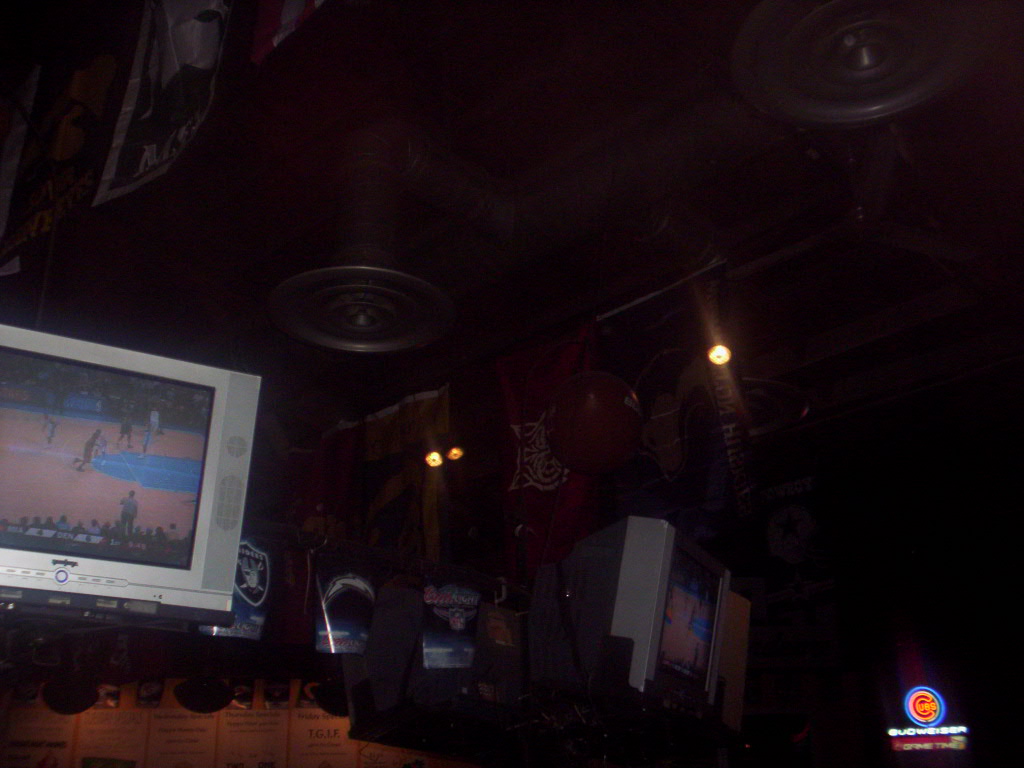The photograph captures a dimly lit scene inside what appears to be a sports bar or memorabilia shop. Dominating the left side of the image is a small, vintage silver TV displaying a colorful basketball game. The wooden gymnasium floor with its large blue design is visible on the screen. Scattered around the TV are various sports memorabilia, including items branded with Raiders and Chargers logos. Despite the pervasive darkness, some small circular lights and a few trinkets can be discerned just to the right of the TV. Another TV or computer screen further to the right also seems to be tuned to a sports game. Flags or banners hang from the ceiling, alongside large round vents. A partially visible neon Budweiser sign, possibly with a "Cubs" mention, adds to the bar-like ambiance. The overall lack of light and clarity makes discerning further details challenging, but the scene unmistakably evokes a cozy, nostalgic sports bar atmosphere.